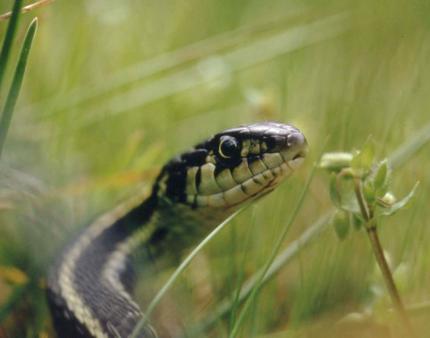This is a detailed close-up photograph of a snake, likely a rattlesnake, slithering through vibrant green grass. The snake, whose visible head and front portion of the body are characterized by black and beige-white (or yellowish) stripes, appears to be of moderate size. The snake has distinct black and green eyes, and it is facing the right side of the frame with a muted expression and closed mouth. Nearby, there is a plant with fuzzy green leaves, possibly a stem or petal of a cotton flower, which stands upright. The blurred background features a field of grass, contributing to the composition without distracting from the snake itself. The image is rectangular in shape and devoid of any text or additional animals, keeping the focus solely on the snake and its immediate surroundings.